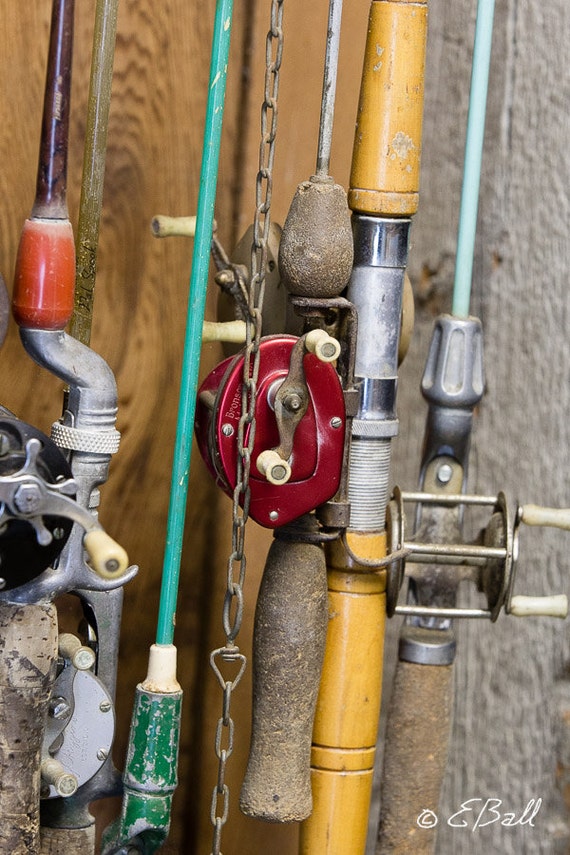This detailed photograph, credited to the photographer with the signature "© EBALL" in script on the bottom right corner, captures an assortment of six well-used and potentially rusty fishing rods of varying colors. The fishing rods, which include hues of dark red, green, yellow, light blue, brown, gray, and deep orange, are propped up against a wooden wall. The focus is on the reels and handles of the fishing rods, showing their aged and somewhat weathered condition. A noticeable detail is a chain running from the top down. The close-up nature of the photo emphasizes the intricate details and textures of the rods and reels, showcasing the craftsmanship and the effects of time on these fishing tools. Some rods lack visible strings and one teal rod extends beyond the frame, highlighting the elongated structure of the poles.